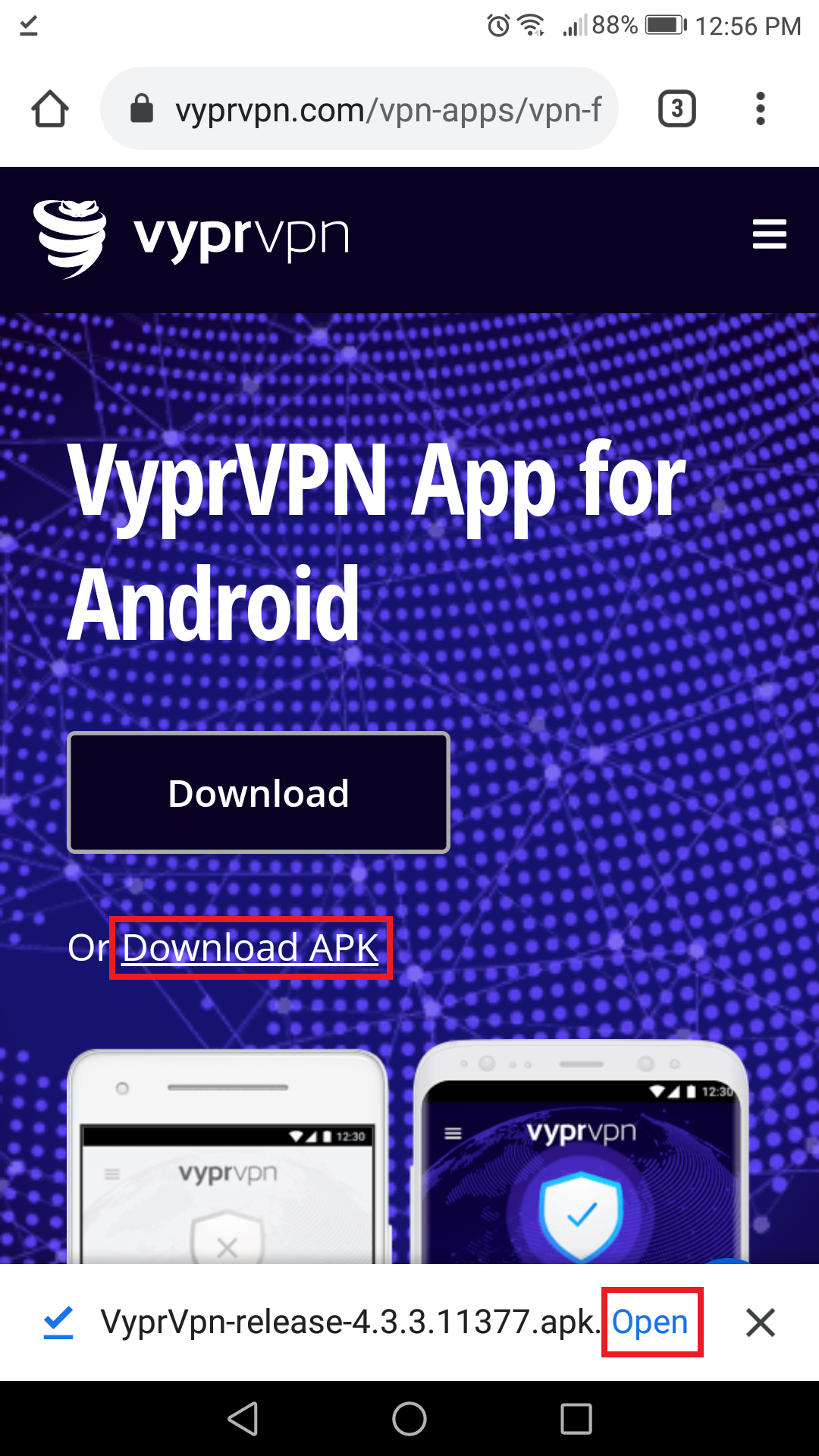In the image, there is a house with a clock set from 12 p.m. to 6 p.m. depicted at the top. The Wi-Fi signal strength is indicated as 3 out of 5 bars, and the battery level is at 88%. The URL displayed is `vpervpn.com/vpn-app/vpn-app-3`. In the center, there is a ViperVPN app interface with a noticeable interconnected pattern of dots and lines. The app offers options to "Download" or "Download APK," highlighted by a red border. 

At the bottom left, there's an image of a white smartphone displaying the ViperVPN shield logo with a checkmark. Adjacent to it, the background is white, displaying "vipervpn shield X." On the right, the text "vipervpn shield checkmark away" is visible, paired with an icon showing full Wi-Fi signal strength. Below this, it reads "vipervpn relay 4.3.3.11.3" with options to send to APK.open. Additional icons including a red-bordered X, a sideways triangle, a circle, and a square are present at the bottom.